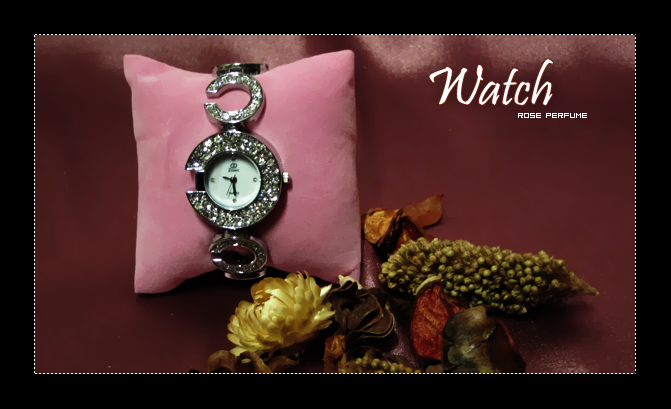This is a detailed photograph of a luxurious watch advertisement. The entire composition is surrounded by a sleek black border, which itself features a white dotted inner border that frames the advertisement. The ad center boasts a sumptuous deep red velvet background, creating an opulent and inviting ambiance.

In the upper right-hand corner of the advertisement, the word "Watch" is prominently displayed in bold white text. Directly beneath it, in a different and elegant font, the words "Rose Perfume" are centered, adding a touch of sophistication and intrigue.

Dominating the left side of the image is a delicate pink pillow, small and tastefully proportionate to the watch it supports. The watch is exquisitely draped around the pillow, showcasing its sparkling gold band. The band elegantly forms the shape of a backward letter "C," with the open part facing the left.

Atop the gold band, there is another band forming a similar backward "C" shape, but in a lighter, shimmering silver hue. Beneath these two bands lies a closed ring, completing the luxurious ensemble.

The watch face itself is unique, lacking full numerals. Instead, it features the word "Zinc" in the upper corner and three dots strategically placed at the left, right, and bottom positions, indicating a minimalist yet refined design.

Finally, beneath the pink pillow and the dazzling watch is an array of flowers. These blooms, though dulled and muted in color, range from soft yellows to greens and oranges, adding a gentle and natural contrast to the striking watch and rich red velvet background. This floral element subtly enhances the ad's overall aesthetic, inviting the viewer to appreciate the exquisite blend of elegance and natural beauty.